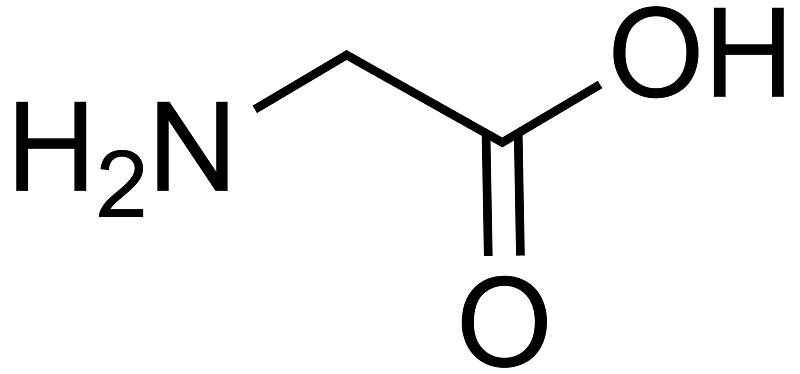The image appears to be a digital illustration of a chemical structure, depicted in black lines and uppercase letters against a plain white background. On the left, the formula begins with "H₂N," where the subscript "2" is positioned slightly lower between the "H" and "N." From "H₂N," a line extends upwards to the right at a 45-degree angle, then zigzags down to the center, leading to a central "O." Two vertical lines drop down from a mid-point in this zigzag line, connecting to the "O" at the bottom center of the image. From the "O," another line angles upwards to the right at 45 degrees, leading to an "OH" positioned in the upper right section. The composition fills the entirety of the rectangular image, providing a clear and structured visual representation of the chemical formula against an otherwise empty white space, emphasizing the black script and lines.